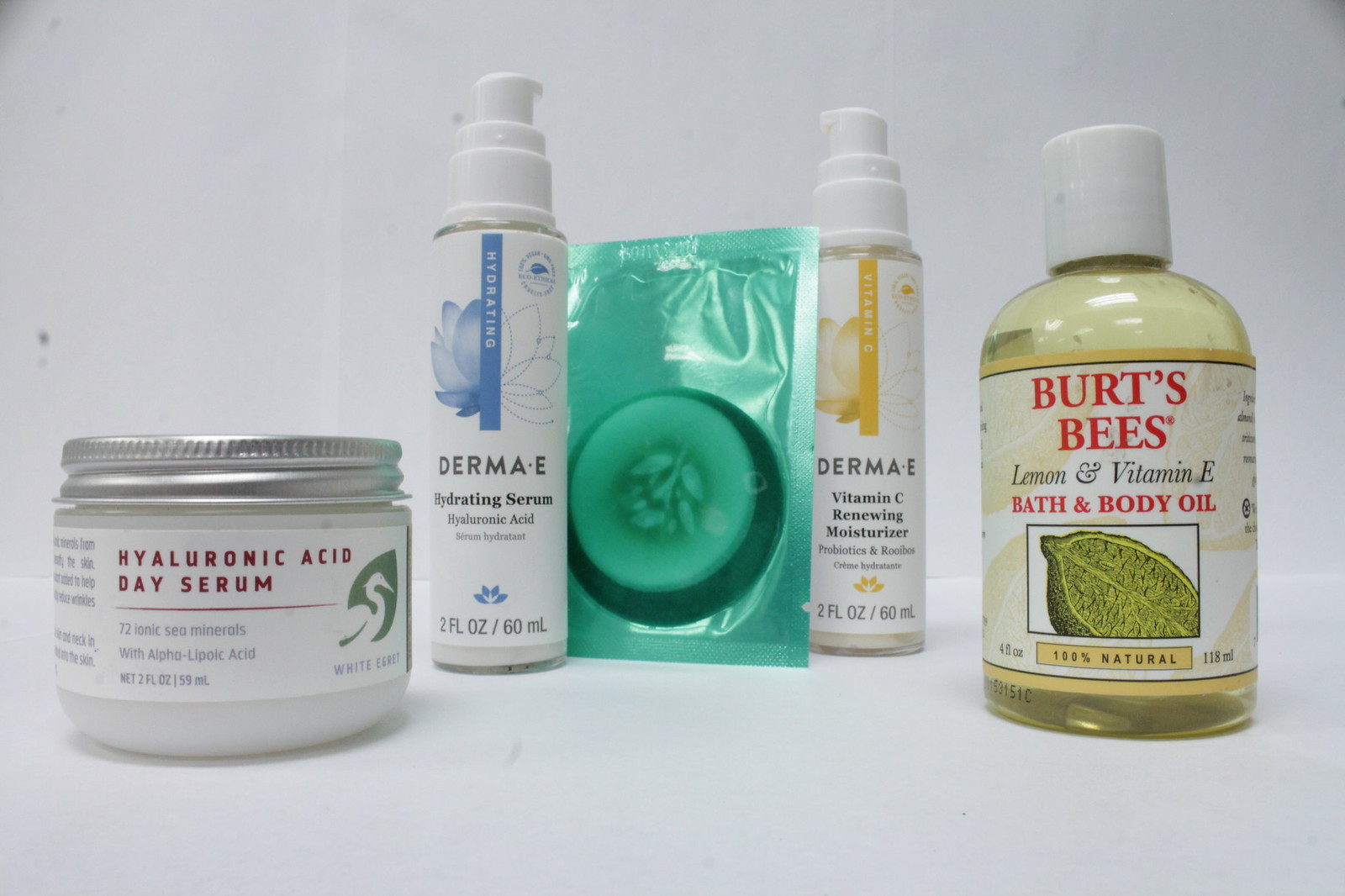The image showcases a neatly arranged collection of five beauty products on a pristine white surface, set against a white wall background. From left to right, the first item is a clear jar with a metal screw cap, prominently labeled in red text on a white background as "Hyaluronic Acid Day Serum." Next, there is a sleek, cylindrical jar topped with a pump cap, branded as "Damai Hydrating Serum." The third product is a circular container wrapped in green plastic, maintaining an air of mystery. Following this, another pump bottle stands, identified by its label as "Damai Vitamin C Renewing Moisturizer." Finally, on the far right, a bottle with a white cap displays the label "BOTS Bees Lemon and Vitamin E Bath and Body Lotion." Each product is distinctly presented, highlighting a curated selection of skincare essentials.